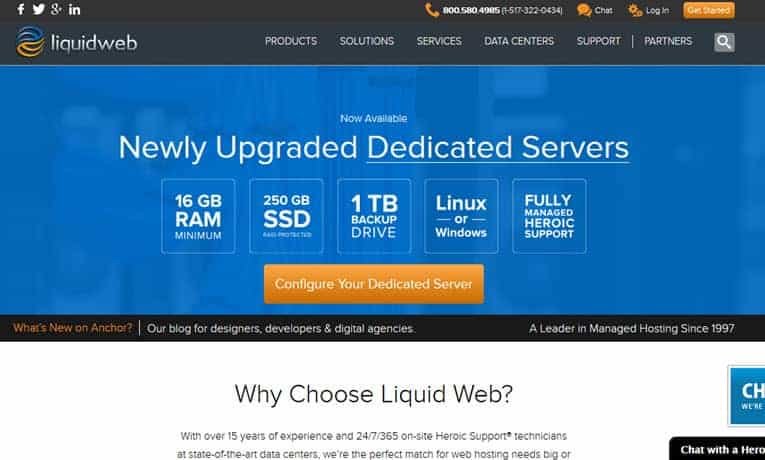Here's a detailed and refined caption for an image, based on the provided description:

"In this image, we see a section of the LiquidWeb company's website, a renowned provider of data centers. The design prominently features the LiquidWeb logo which includes both blue and orange swirls, with 'LiquidWeb' written in white above the logo. On the black background header, there are several social media symbols: Facebook, Twitter, Google+, and LinkedIn, all in white. The navigation menu includes headings for Products, Solutions, Services, Data Centers, Support, and Partners.

There is also a white magnifying glass icon within a gray box, and above this, an orange button labeled 'Get Started.' Another orange feature includes gears next to the 'Login' text, and speech bubbles beside 'Chat.' Additionally, a phone icon is present with the numbers 800-580-9485 and (517) 322-0434 in parentheses.

In the main section, set against a dark blue background with white text, the focal announcement reads, 'Now Available: Newly Upgraded Dedicated Servers,' with 'Dedicated Servers' underlined. Below, five boxes specify features: '16GB RAM Minimum,' '250GB SSD,' '1 Terabyte Backup Drive,' 'Linux or Windows,' and 'Fully Managed Heroic Support.' There is an orange button with white text labeled 'Configure Your Dedicated Server.'

At the bottom, another black bar highlights 'What's New on Anchor,' and leads to a blog intended for designers, developers, and digital agencies. In the bottom right corner, the tagline reads, 'A Leader in Managed Hosting Since 1997.'

The very bottom of the page is somewhat cut off but includes a partial message promoting LiquidWeb's 24/7/365 on-site heroic support at state-of-the-art data centers. Adjacent to this message is an orange button labeled 'Chat with a Hero.' Another section above shows a blue background with part of the phrase 'CH' and 'we're,' although it is also partially cut off."

This revised caption offers a thorough and structured description of the image, retaining all key details.